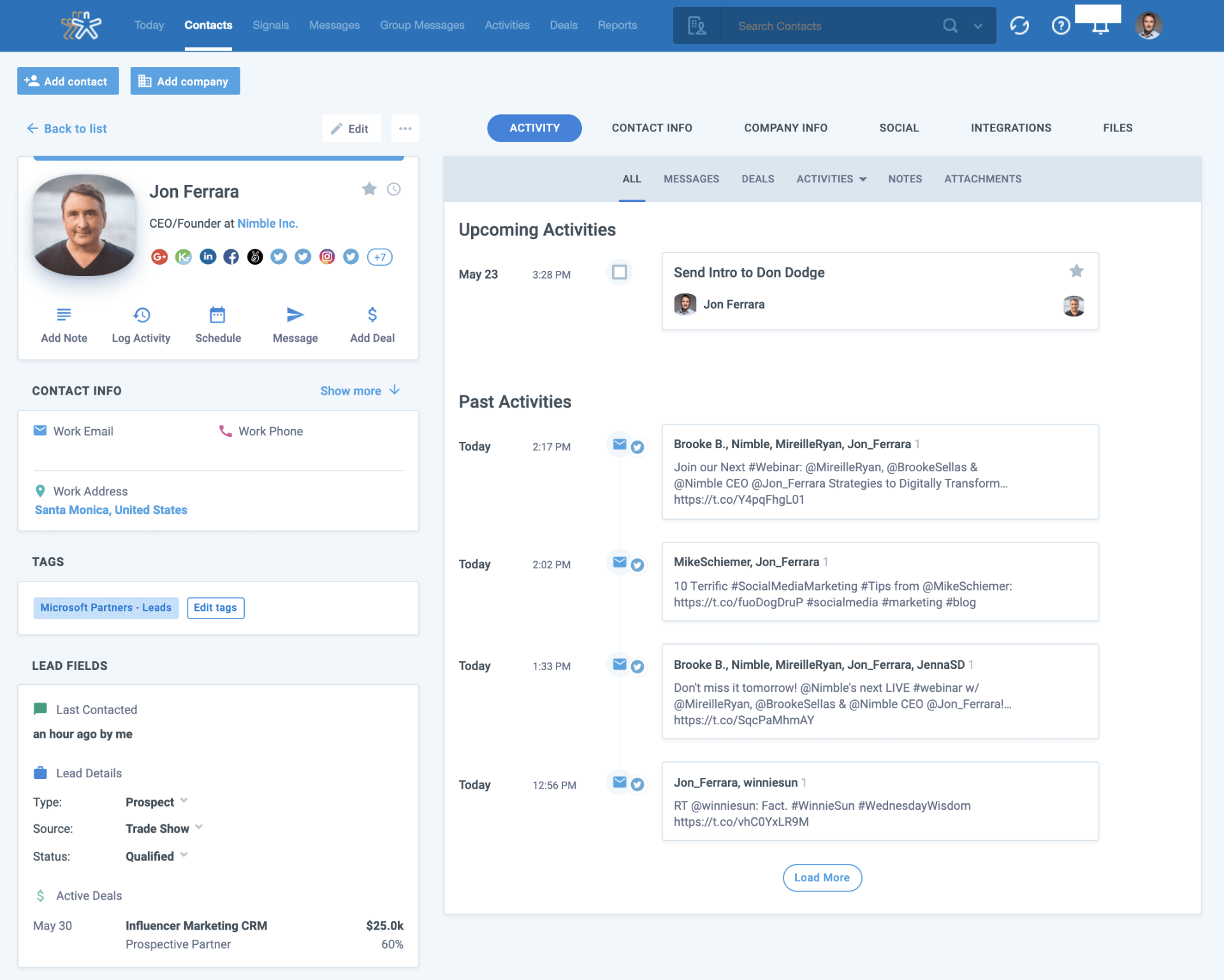**Caption:**
The image appears to be a detailed profile dashboard for a user named John Ferreira, CEO and Founder of Nimble Inc. At the top of the dashboard is a blue navigation bar with tabs labeled "Today," "Contacts," "Signals," "Messages," "Group Messages," "Activities," "Deals," and "Reports." Accompanying these tabs is a search bar and several icons at the upper right, including a profile icon.

Below the navigation bar, there are two action buttons labeled "Add Contact" and "Add Company." John Ferreira’s profile information is prominently displayed, including his title and a picture of him. 

On the right side of the dashboard, there are multiple navigation options for different sections which include "Activity" (highlighted), "Contact Info," "Company Info," "Social Integrations," and "Files."

The "Activity" section provides a detailed view of John Ferreira’s engagements. It is divided into two parts: "Upcoming Activities" which lists tasks such as "Send intro to Don Dodge" along with the date, and "Past Activities" which includes a log of multiple emails sent on the same day.

On the left side of the dashboard is the "Contact Info" section displaying John's work email, work phone, and work address. Below this section, there are categories for "Tags" and "Lead Fields," which offer insights into various lead deals including the type, source, and status of each deal.